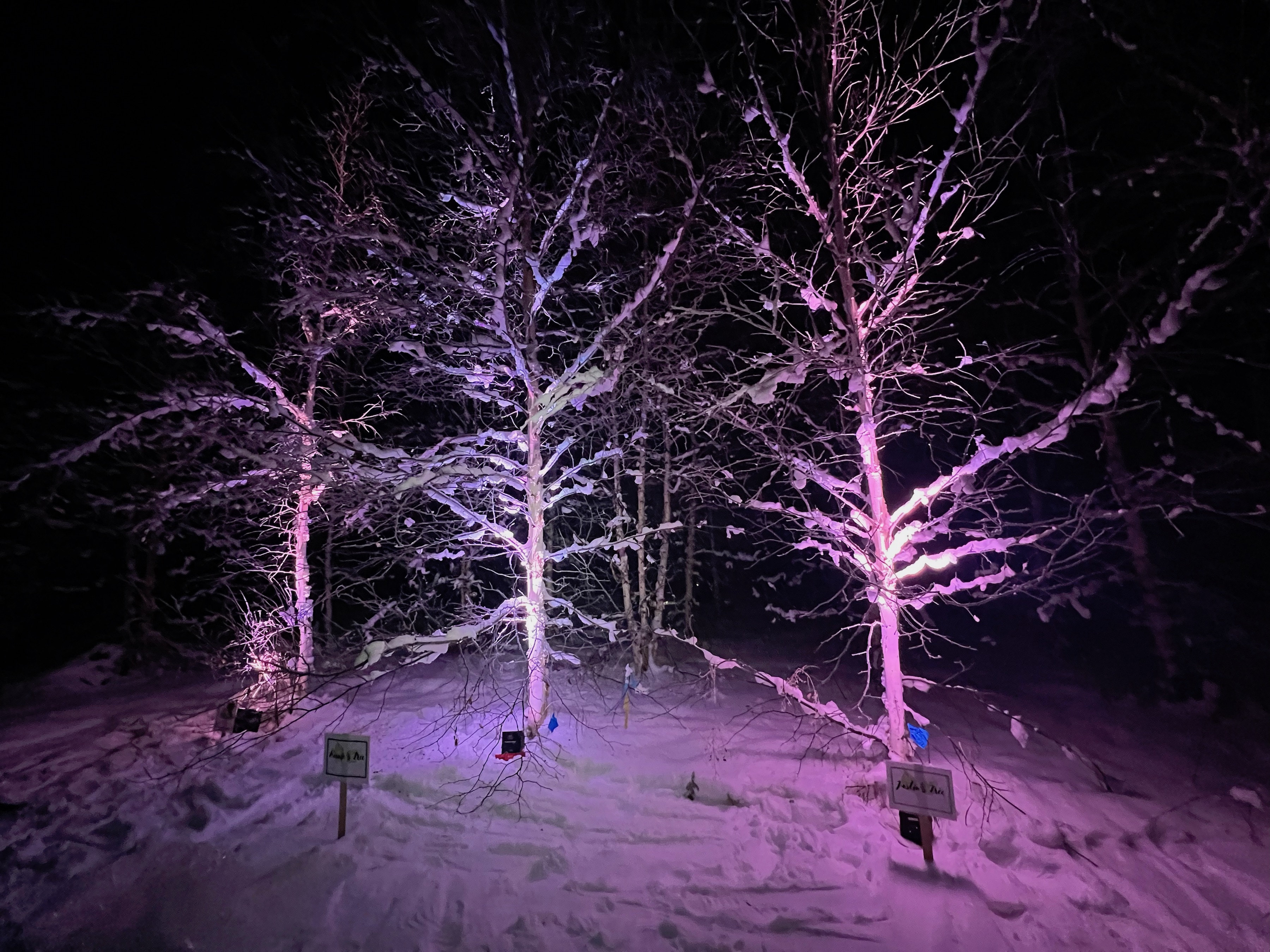This nighttime landscape photograph captures a serene, snow-covered scene dominated by three bare trees positioned left, center, and right. The trees' branches are heavily laden with snow and are elegantly highlighted by landscape lighting, which casts a white hue on the central tree while bathing the outer trees in a subtle purple glow. The surrounding ground is also covered in snow, marked with numerous footprints, evidencing recent activity. In front of the trees, two small, legible signs with wooden stakes and white boards edged in black stand out against the snowy terrain. The backdrop reveals a solid black sky and more distant, obscured trees, suggesting an expansive, cold environment. The photograph, with its vivid purple, white, and black contrasts, provides a strikingly clear and realistic snapshot of this wintery outdoor setting.